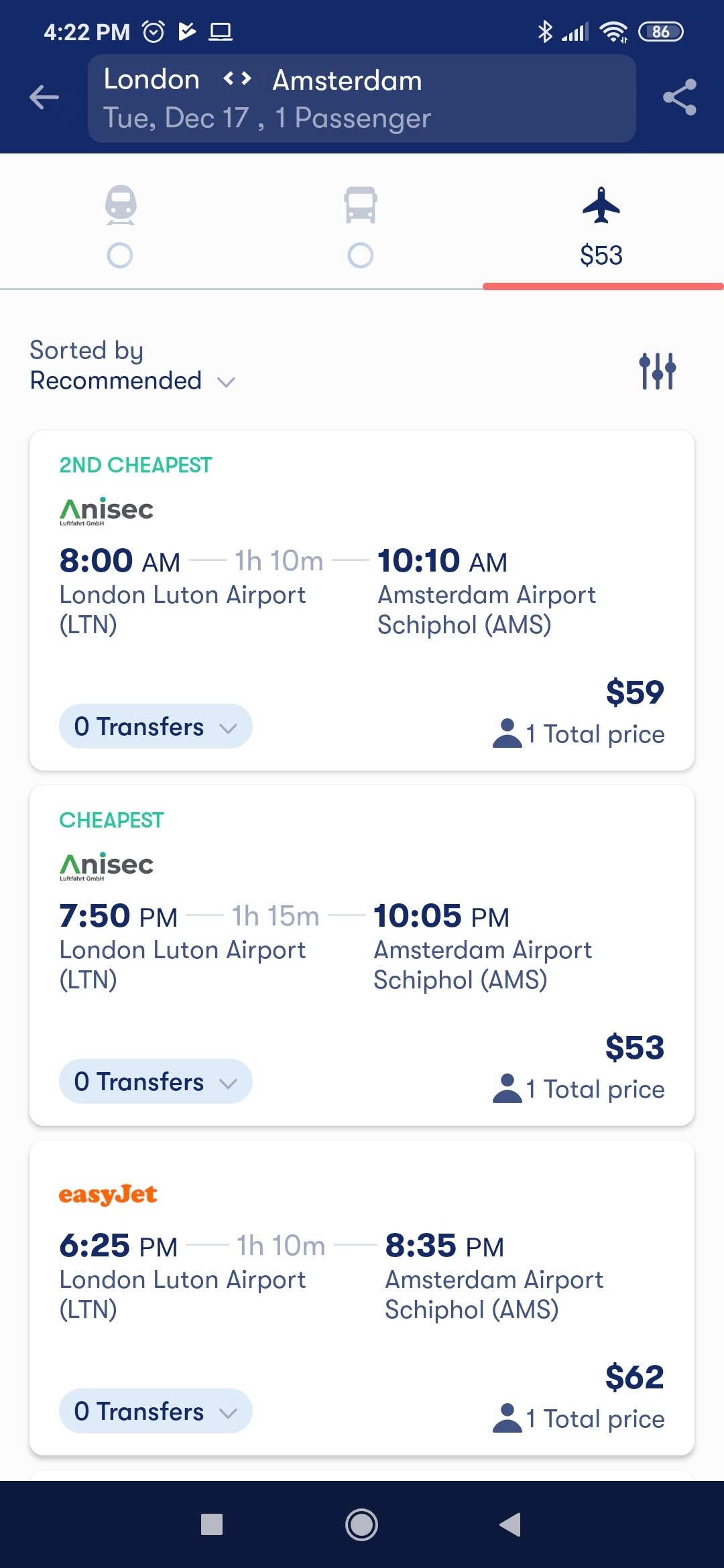**Flight Itinerary Screenshot: London to Amsterdam**

In this screenshot of a flight itinerary, the top header is a rich navy blue. Within the header, at the top left corner, the time reads 4:22 PM accompanied by icons of an alarm clock and a laptop. On the right side, a battery status indicates 86% charge. The header also includes key details about the flight: the journey is from London to Amsterdam, scheduled for Tuesday, December 17, with one passenger.

Below the header, the website background shifts to white. Directly under the header, three icons are displayed in a horizontal row: a train icon, a bus icon, and a flight (airplane) icon in blue. The flight icon, underlined in pink, shows a fare of $53.

Underneath this row of icons, the page is divided into three sections, each detailing different flight options. The page is titled "Sorted by: Recommended."

1. **First Option (Second Cheapest)**
   - Airline: Anisec
   - Departure: 8:00 AM from London Luton Airport
   - Arrival: 10:00 AM at Amsterdam Airport
   - Cost: $53 per person

2. **Second Option**
   - Airline: Anisec
   - Departure: 7:50 PM from London Luton Airport
   - Arrival: 10:05 PM at Amsterdam Airport
   - Cost: $53 per person

3. **Third Option**
   - Airline: EasyJet (highlighted in orange)
   - Departure: 6:25 PM
   - Arrival: 8:35 PM
   - Duration: Approximately 1 hour and 10 minutes
   - Transfers: None
   - Cost: $62 per person

This detailed breakdown provides a comprehensive view of the available flights, helping the traveler make an informed choice.